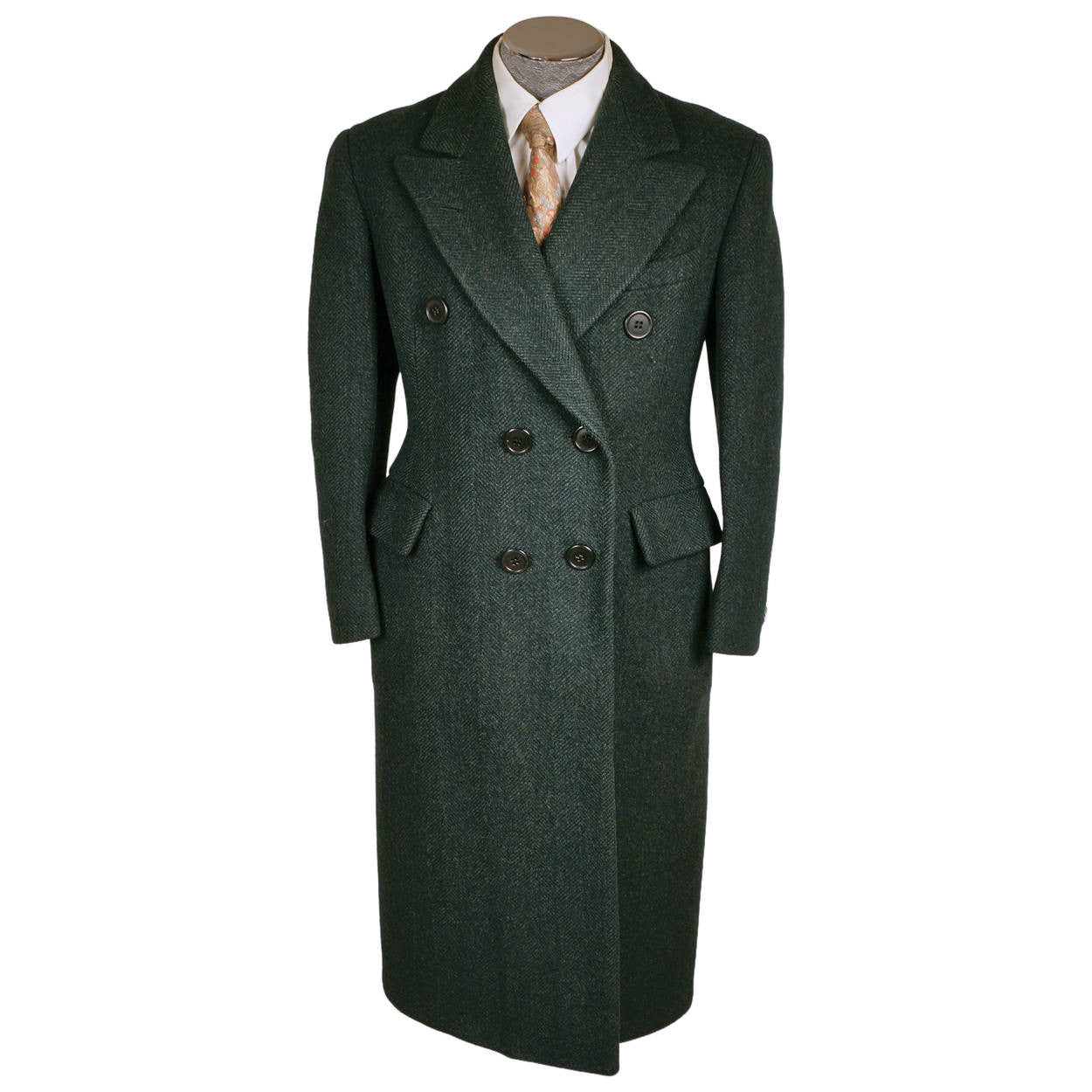This full-color, vertically rectangular photograph, taken for marketing purposes, features a headless mannequin displaying an elegant ensemble. The mannequin has no arms or legs, only showcasing its torso and neck. It is dressed in a sophisticated, double-breasted overcoat made of tweed material, in a dark gray or possibly navy blue color. The coat, which appears to be tailored for a masculine fit, prominently features six black buttons, with four functional buttons securing the coat and two additional decorative buttons positioned near the chest area. Two front pockets are visible at the waist level of the coat. Underneath the overcoat, the mannequin wears a white dress shirt, potentially adorned with faint gray diagonal stripes, paired with an ornate tie. The tie, while primarily a copper or brownish-orange color, hints at pink and peach accents, adding a touch of flair to the formal attire. The entire scene is set against a plain white background, emphasizing the meticulously coordinated outfit.